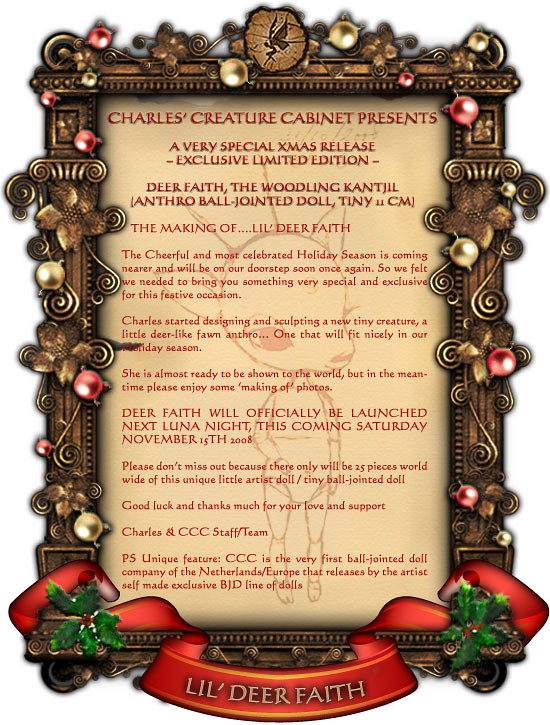In this exclusive and intricately designed Christmas-themed message, a beautifully ornate, bronze-colored frame adorned with pearls, holly sprigs, and a red ribbon encases the heartfelt announcement. The frame, reminiscent of medieval artistry, features delicate vine-like trails culminating in detailed holly leaves and red berries at the bottom corners. The message, accentuated with festive elements and a digital sketch of an enchanting little fawn-like creature with a human body and large, expressive eyes, reads: "Charles Creature Cabinet Presents a Very Special Xmas Release Exclusive Limited Edition." It introduces "Little Deer Face," a unique, handcrafted ball-jointed doll designed by Charles and his team. This limited edition doll, just 25 pieces worldwide, promises to enhance the cheer of the most celebrated holiday season. It highlights the dedication of the CCC, the pioneering ball-jointed doll company in the Netherlands and Europe. With a P.S. mentioning the Netherlands, this detailed digital artwork invites doll enthusiasts to anticipate the official launch on November 15th, 2008, while enjoying behind-the-scenes photos of "Little Deer Face."